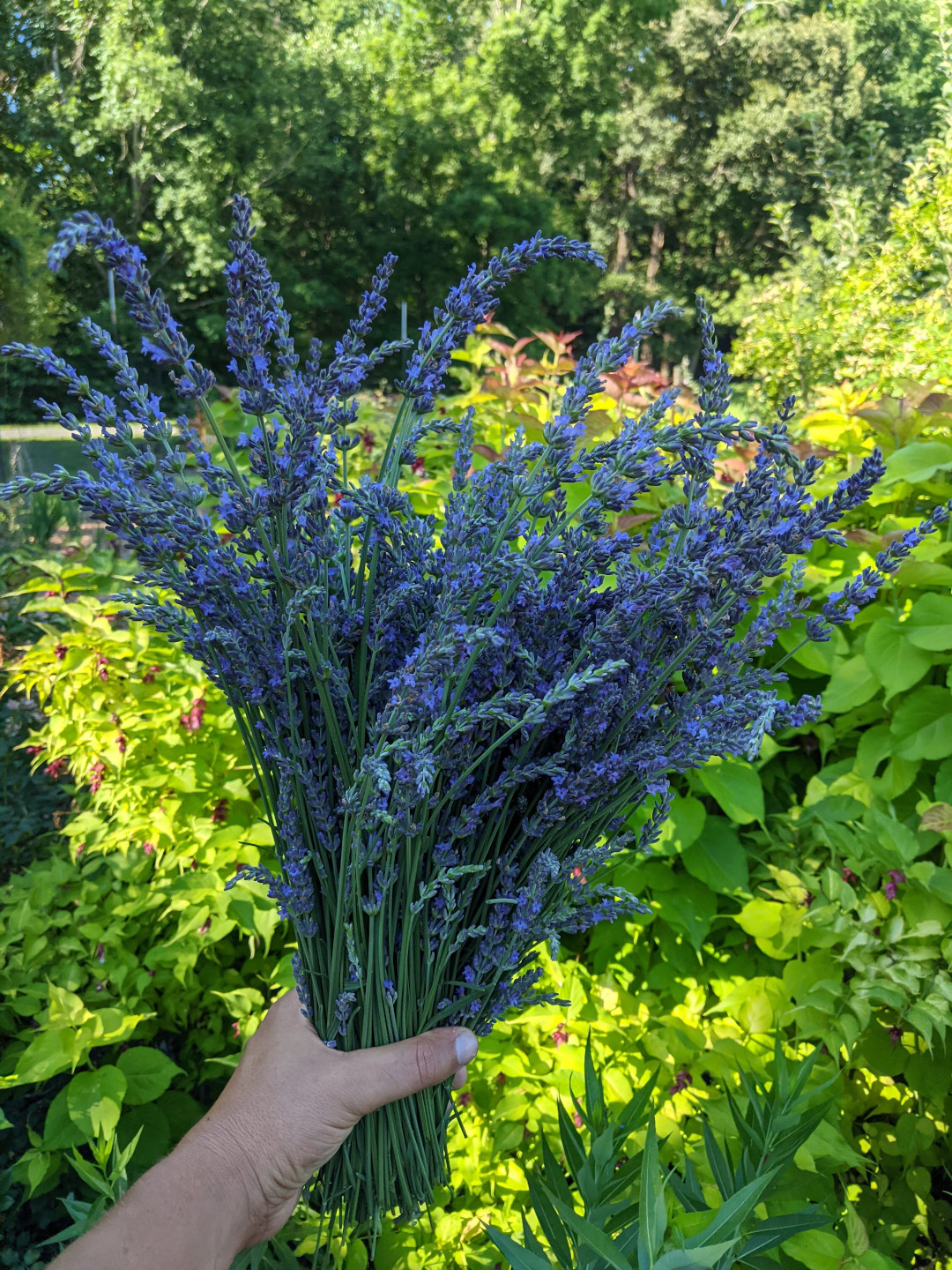This photograph captures a lush, outdoor scene abundant with greenery. The background is filled with various-sized trees and bushes, creating a richly textured, verdant setting illuminated by sunlight. Foreground details dominate the composition, where a hand—likely a man's but with debated gender due to imagery—extends from the bottom left corner, holding a freshly cut bunch of lavender that boasts strikingly beautiful purplish-blue flowers. The hand, adorned with white nail polish, presents the lavender directly to the camera, making it the focal point of the image. The lavender contrasts vividly with the surrounding vibrant greens and adds a touch of delicate beauty. Additionally, some reddish flowers are scattered among the bushes in the background, contributing more color variety to the scene. This picturesque setting, possibly in a backyard, evokes a sense of tranquility and natural beauty, reminiscent of similar aesthetically pleasing images frequently shared on social media.